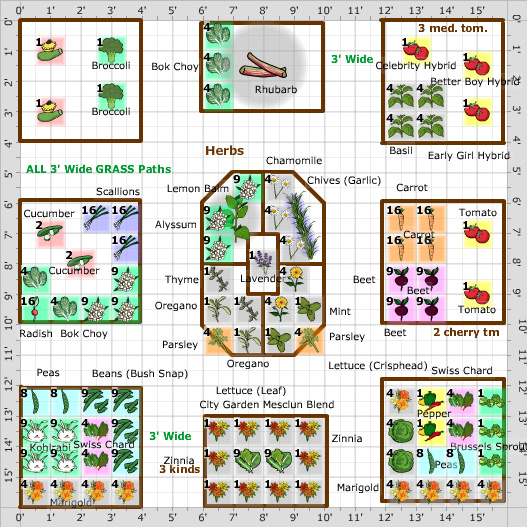The image is an intricately detailed garden plan depicted on a grid, with each axis marked from zero to 15 feet, demarcating precise spatial segments. Various rectangular and polygonal areas within this grid outline the proposed sections for different plants and vegetables.

In the top-left section, there's broccoli along with gourds. The center-top area contains bok choy and rhubarb, while the top-right is designated for hybrid tomatoes and basil. The middle-left area features scallions, cucumber, bok choy, and radish. Dominating the middle of the grid is an octagonal section dedicated to a variety of herbs including thyme, oregano, parsley, lavender, chamomile, chives, mint, allicin, and lemon balm.

Moving to the center-right of the grid, there's a section for carrots, beets, and cherry tomatoes. The bottom-left is plotted for growing peas, beans, Swiss chard, and marigolds. The center-bottom area is reserved for lettuce, zinnia, and potentially mesclun mix. Finally, the bottom-right section is allocated for peppers, Brussels sprouts, peas, and additional marigolds.

Running throughout the grid, three-foot-wide grass pathways provide access to each planting section, ensuring ease of movement and maintenance within the garden. This thoughtfully created garden chart captures a comprehensive plan for a diverse array of vegetables, herbs, and flowers.